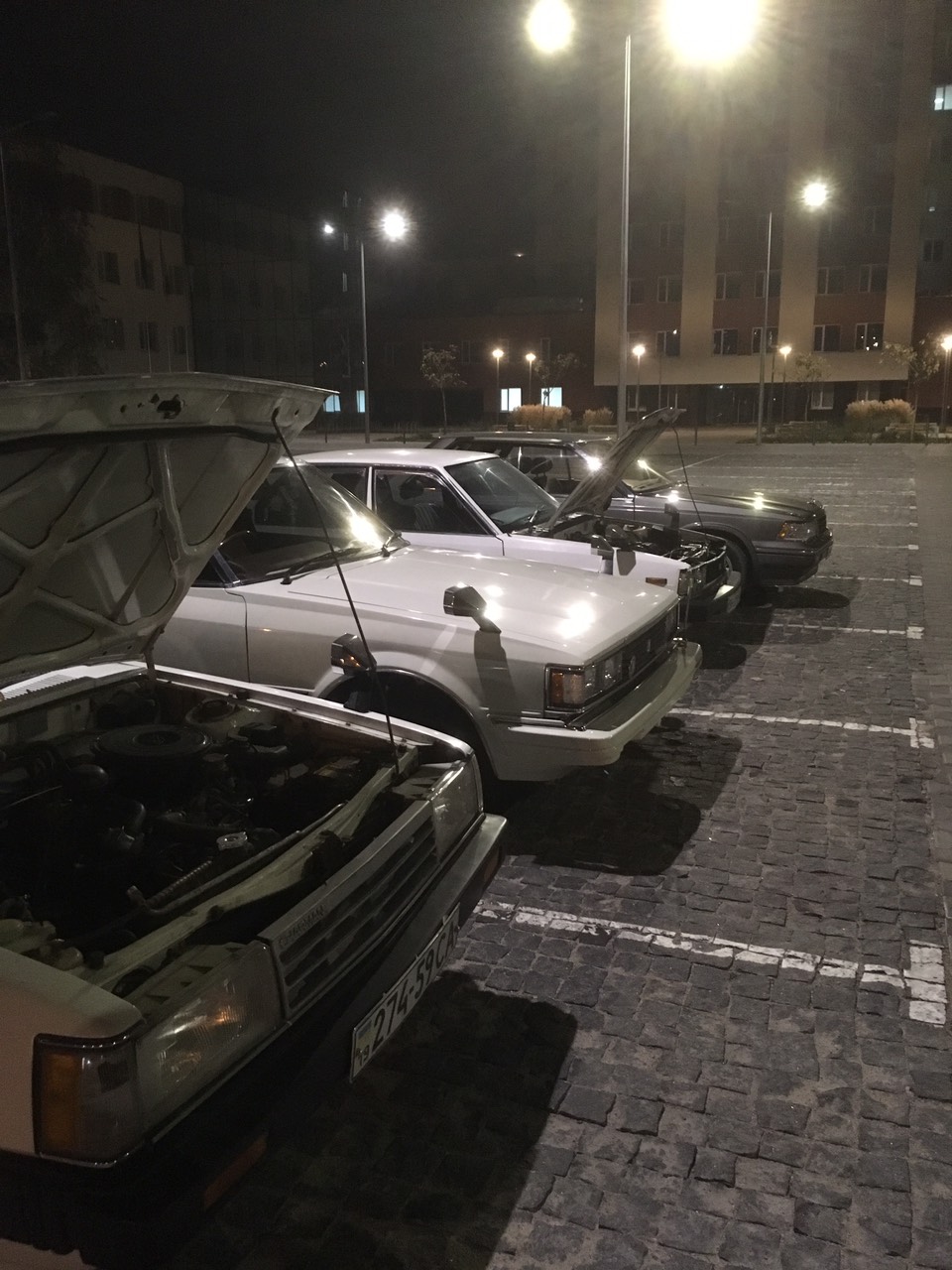In this nighttime image, we see a sequence of four older cars parked diagonally in a cobblestone parking lot, with the perspective starting from the closest car extending into the background. The nearest car, with its hood up, prominently displays a mostly legible front license plate reading "27459CA." Adjacent to it is a white sedan with its hood down, followed by another white sedan with its hood up, both exhibiting a boxy design typical of late 80s models. The farthest car is a gray, similarly aged sedan with its hood down. In the background, several empty parking spaces lead to buildings that suggest a school campus. Street lamps illuminate the scene with a muted light, adding a subtle glow to the cobblestone ground marked by white parking lines. The overall monochromatic tone nearly mimics a black-and-white photograph.